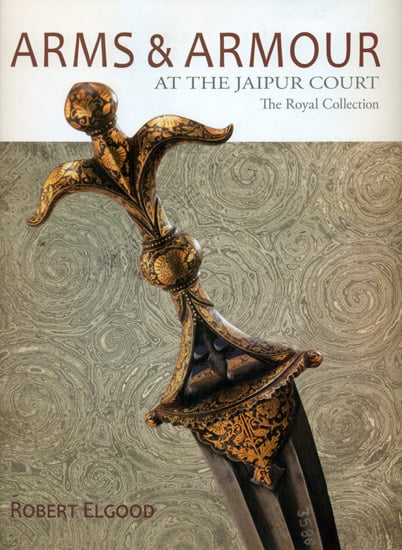The cover of the book "Arms and Armor: At the Jaipur Court – The Royal Collection," authored by Robert Elgood, prominently features an ornate sword. The title, "Arms and Armor," is displayed at the top in bold brown lettering, followed by smaller gray text that reads "At the Jaipur Court," and even smaller text below it that states "The Royal Collection." The typography is right-justified on a white background, while the rest of the cover displays a sand-colored texture with intricate swirl patterns. Dominating the cover is the image of a gold or brass sword handle adorned with a fleur-de-lis pattern, oriented diagonally from the top left to the bottom right. We also see the point where the handle meets the blade, which is black in color, although the entire blade is not visible. In the lower-left corner of the cover, the author's name, Robert Elgood, is printed in bold.